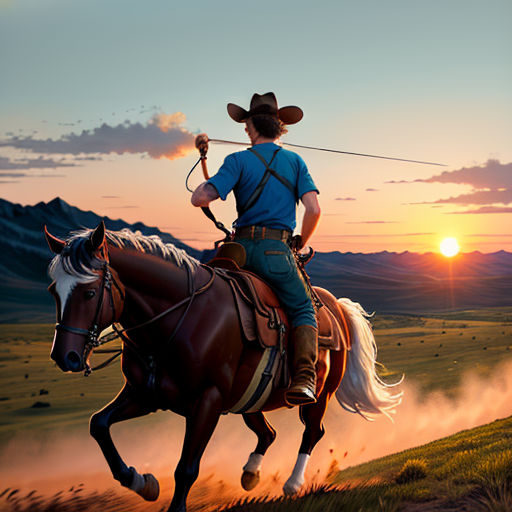In this whimsical and animated-styled painting, a cowboy wearing a blue short-sleeved shirt, blue jeans, a belt, brown leather boots, and a traditional cowboy hat is humorously portrayed riding a brown horse with a white mane, white tail, and white sock feet. Unusually, the cowboy is seated backwards on a brown saddle, his back facing the horse's head while his feet point forward in the stirrups. The horse, adorned with a white star on its forehead, gallops to the left, kicking up dirt and grass as it runs across a prairie setting. The scene is set against a picturesque backdrop of a sunset to the right, casting an idyllic light over the landscape with mountains in the distance, a blue sky scattered with clouds, and the dust rising from the horse's hooves. The cowboy is seen throwing a lasso or rope, adding to the dynamic and whimsical nature of this piece.